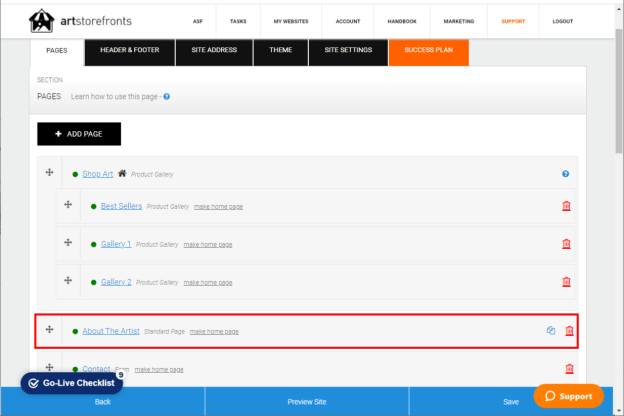This color screenshot, appearing to be taken from a website, prominently features a small black-and-white tent icon at the top, representing the "Art Store France." The text next to the icon is blurred and unreadable, even when zoomed in to 214%. However, key menu items, such as "Account," "Annotation," "Marketing" (highlighted in orange), and "Sport," are visible. 

Below this section are several navigation tabs labeled "Pages," "Books," and "Ticked." Additional tabs in black are labeled "Header and Footer," "Site," "Address," "Theme," "Site Settings," and "Success Plan." The next section titled "Pages" includes a guide labeled "Learn how to use this page," marked by a blue dot. 

A prominent black button labeled "Add Page" in white text, accompanied by a plus sign, is visible. There are also links labeled "Shop Art," "Best Sellers," "Gallery 1," and "Gallery 2." The link "About the Artist" is highlighted with a red rectangle. Below this, obscured by a "Go Live Checklist" button in dark blue with white text, is an unreadable item.

At the bottom of the image, there are three blue panels with white text: "Back," "Preview Site," and "Save." In the bottom right-hand corner, an orange curved rectangle with "Support" written in white, accompanied by a voice bubble icon, is visible.